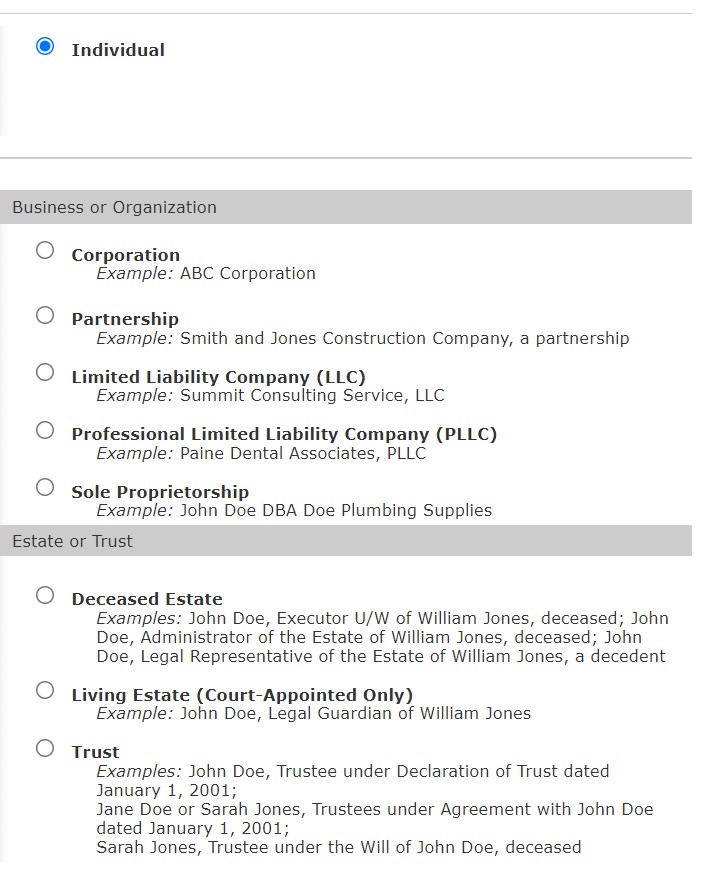The image showcases a user interface screen that appears to be part of an online form or application related to selecting an entity type. 

At the top of the screen, the word "Individual" is prominently displayed and highlighted with a blue dot, indicating it has been selected. Wide expanses of white space create a clean, minimalist layout. Below the selected "Individual" option, a grey bar presents the heading "Business or Organization."

Under this heading, several options are listed, each with an accompanying, but unselected, grey dot:
- Corporation
- Partnership
- Limited Liability Company
- Professional Limited Liability Company
- Sole Proprietorship

Further down, another heading labeled "Estate or Trust" lists additional options, each also marked by an unselected grey dot:
- Deceased Estate
- Living Estate
- Court Appointed Only
- Trust

Each category is followed by examples to clarify the entity types. For instance, "ABC Corporation" under "Corporation" and "John Doe, Legal Guardian of William Jones" under "Living Estate."

The overall design focuses on providing clear choices while leaving ample space for readability.